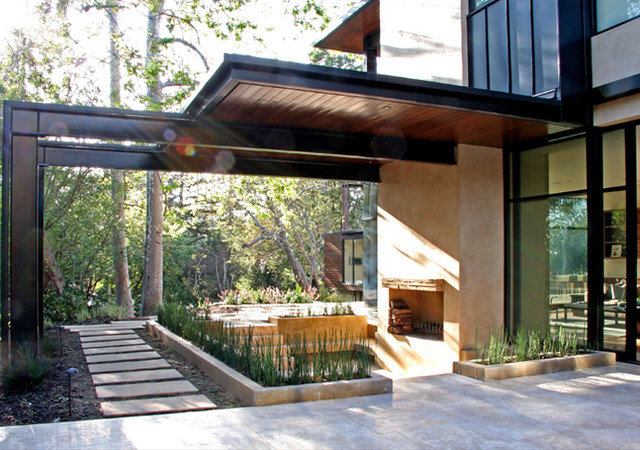This photograph captures the exterior of a highly modernistic, multi-story house, characterized by extensive use of glass walls and large windows. The house, present in the right side of the image, features a sleek design with squared edges and a mix of materials including metal, stone, and wood. A prominent feature is the black-edged awning with wooden planks running underneath, creating a sophisticated porch covering. The outdoor area in the foreground showcases gray concrete flooring and long concrete planters filled with grass and various plants. Additionally, there is a stone walkway composed of separate cement steps or long pavers leading to an entryway under the awning. An outdoor fireplace, yet to be used, is a focal point, complemented by a neatly stacked firewood holding area cut into the house's side. Surrounding the property is a lush, wooded area with large trees and abundant greenery, basking in sunlight that beams from the top left corner on this bright, sunny day. The sky above is a light shade, enhancing the serene atmosphere of this modern architectural setting.